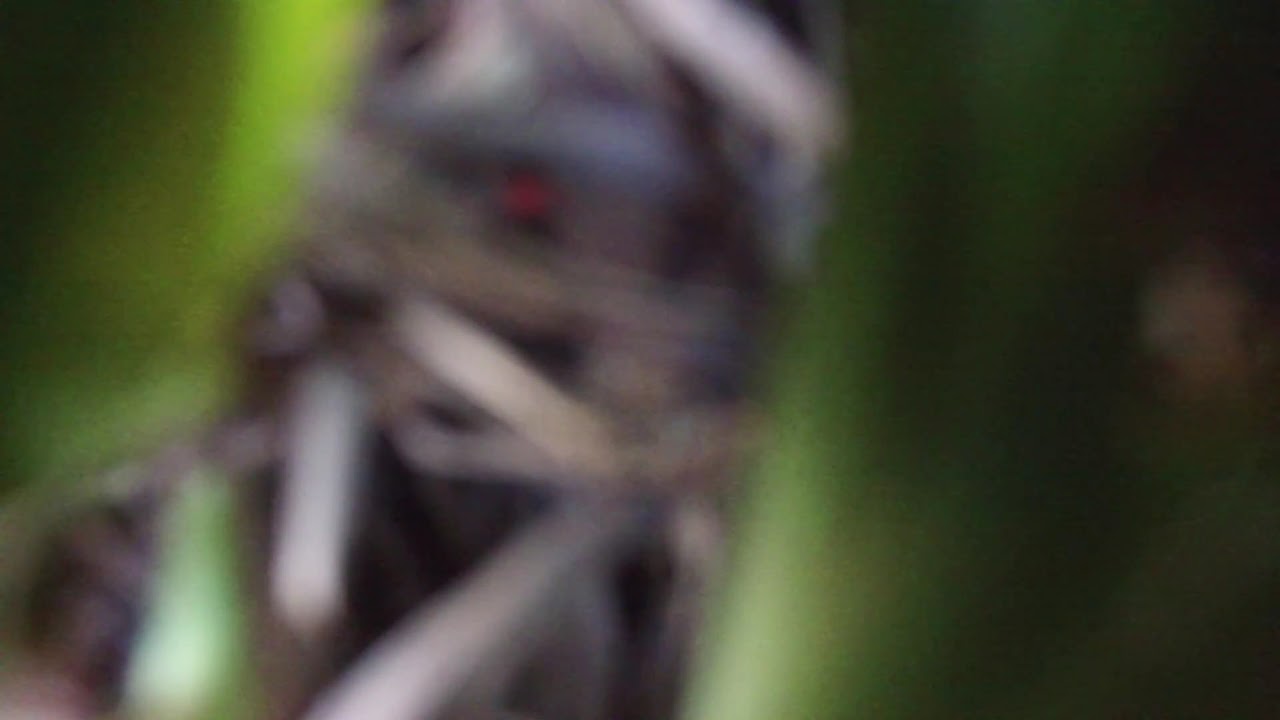The image is extremely blurry and challenging to decipher, but certain elements can be discerned with some consistency across the descriptions. The center of the image contains a dark object that is predominantly black, with white and gray areas and a noticeable red dot that could be perceived as an eye. This central figure has features that evoke a robotic mummy with bandages or wrappings, suggesting a humanoid shape. The surroundings are primarily green, implying an outdoor setting with plants or trees, giving a sense of being in a jungle or heavily vegetated area. Other interpretations hint that this could possibly be a close-up of an insect, a dog, or even a figure lying in a hammock, though the overwhelming blur makes it difficult to draw any definitive conclusions about the exact nature of the subject.